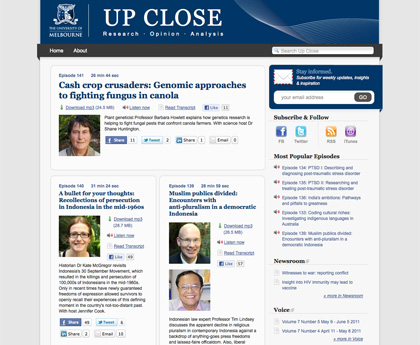A detailed and cleaned-up caption for the image:

"This is a screenshot of a website, likely affiliated with the University of Melbourne, featuring an online newsletter or news portal titled 'Up Close.' The page prominently displays three main articles that cater to a diverse range of academic interests. The first article, titled 'Cash Crop Crusaders: Genomic Approaches in Fighting Fungus in Canola,' includes a small image of the author and appears to delve into cutting-edge agricultural research. The second article, 'A Bullet for Your Thoughts: Recollections of Persecution in Indonesia in the Mid-1960s,' presents a woman's personal reflections and historical analysis of political oppression. The final featured article, 'Muslim Publics Divided: Encounters with Anti-pluralism and Democratic Indonesia,' authored by two individuals, explores the complexities and challenges of pluralism in Indonesian society. The sidebar includes links to other popular updates, episodes, and a podcast, offering additional in-depth content on a variety of subjects."